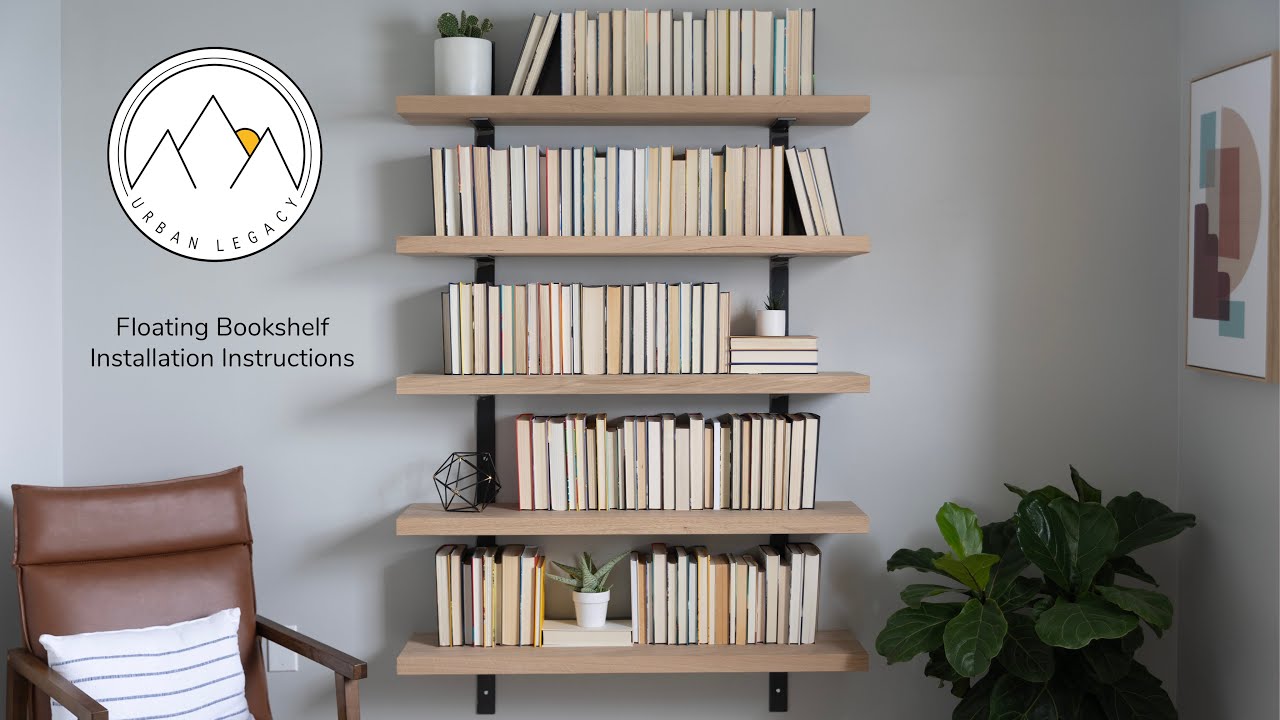The interior of the room features light gray walls and a bookcase centrally positioned as the focal point. This bookcase, characterized by its light wood shelves and black supports, is mounted on the wall and contains five rows laden with books and a few small potted plants. A prominent element in the space is the white Urban Legacy logo with black text, depicting three mountains and the sun, captioned "Floating Bookshelf Installation Instructions" in black, located in the upper left corner. 

To the left of the bookcase, a brown leather armchair with a medium shade back and a white pillow adorned with thin black stripes adds a cozy touch. On the right, the wall displays a framed artwork with a white background that features abstract shapes in tan, light red, brown, and light blue hues. Nestled in the corner between the bookcase and the artwork, a small green leafy plant adds a touch of nature. Additionally, a larger potted plant casts a shadow from the bottom right corner, anchoring this meticulously arranged space.